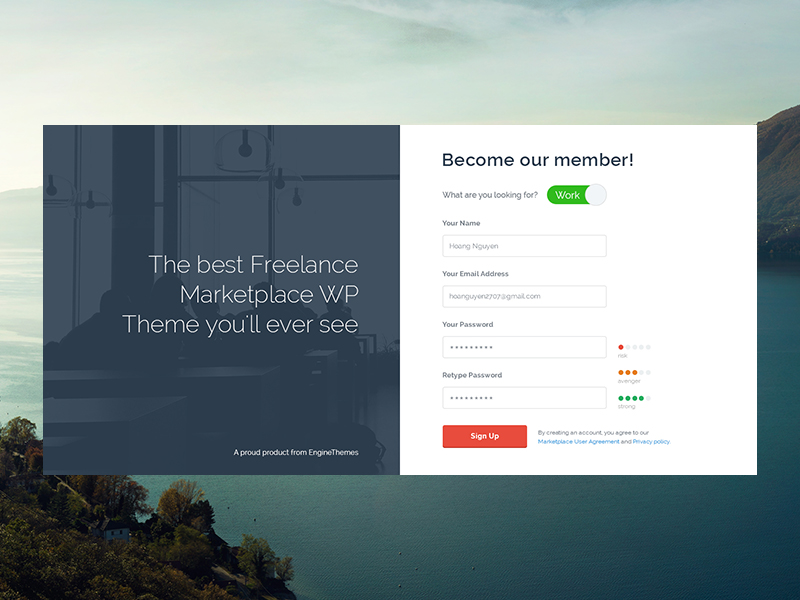A screenshot of a signup page for a freelance marketplace website featuring a visually engaging theme. On the left side, bold text declares "The Best Freelance Marketplace WP Theme You'll Ever See," overlaying an indistinct background image. On the right side, the page invites users to "Become Our Member," prompting them with the question, "What are you looking for?" A toggle option is set to "Work." Below this, there are input fields for "Your Name," "Email Address," "Password," and "Retype Password."